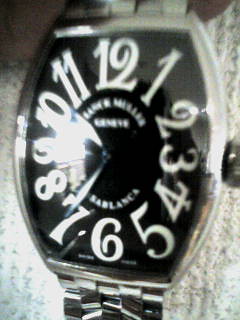The image depicts a woman's watch, characterized by its distinctive and elegant design. The face of the watch is a softly rounded rectangle with a black background, adorned with large, decorative white numbers in a curly, script-like font, reminiscent of a Betsy Johnson style. The numbers 1 through 12 are displayed prominently, and additional small, white letters curve subtly around the top and bottom of the watch face, though they are blurred and unreadable. Notably, the long hand points to the 7, while the short hand rests between the 10 and 11 marks. The watch case and band are made of stainless steel, with a crisscross checkered pattern, adding a touch of sophistication. The watch's knob for time adjustment is visible on the side. The overall image quality is low and somewhat blurry, making finer details harder to distinguish. The watch is positioned on a textured, gray and white tweed fabric that appears to have slight speckling of green and pale purple, adding depth and contrast to the presentation.